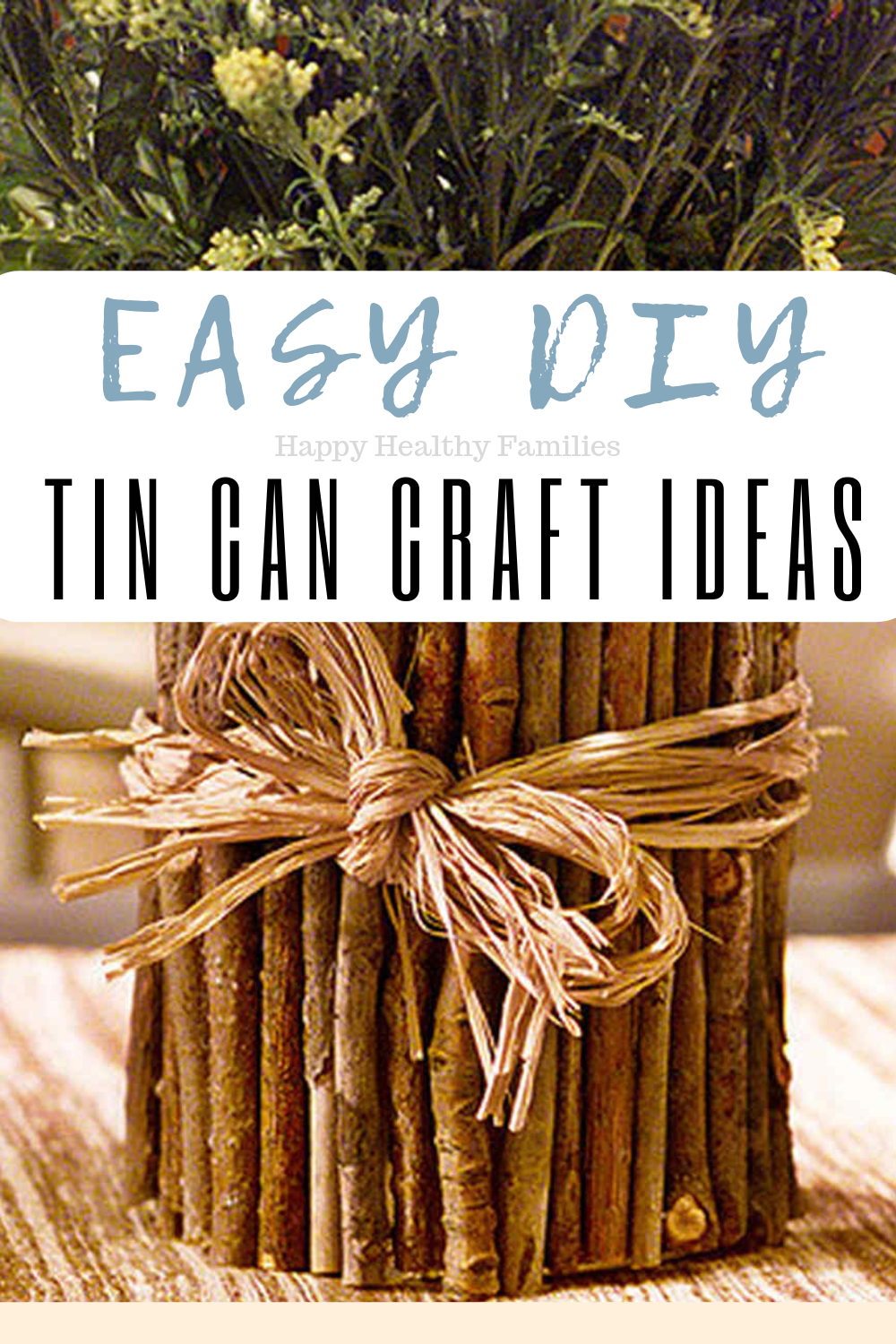This image appears to be a banner or header from a craft blog, possibly the cover of a magazine or book. The focal point is a DIY planter, featuring a tin can that has been creatively transformed into a vase by gluing a bundle of brown twigs around it, which are secured with a pinkish-tan raffia bow. The top of the planter showcases a collection of green leaves and stems, possibly baby's breath, interspersed with small yellow and orange flowers. The entire composition is set on a table with a brown and beige placemat or throw rug as the base. 

A white banner with a peach background overlays the middle of the image. In blue text, it prominently displays "EASY DIY," followed by "HAPPY HEALTHY FAMILIES" in light gray letters and "TIN CAN CRAFT IDEAS" in large black capital letters. The image is bright and close-up, though the resolution is somewhat low, emphasizing the detailed craftwork despite some areas being blocked by the text banner.